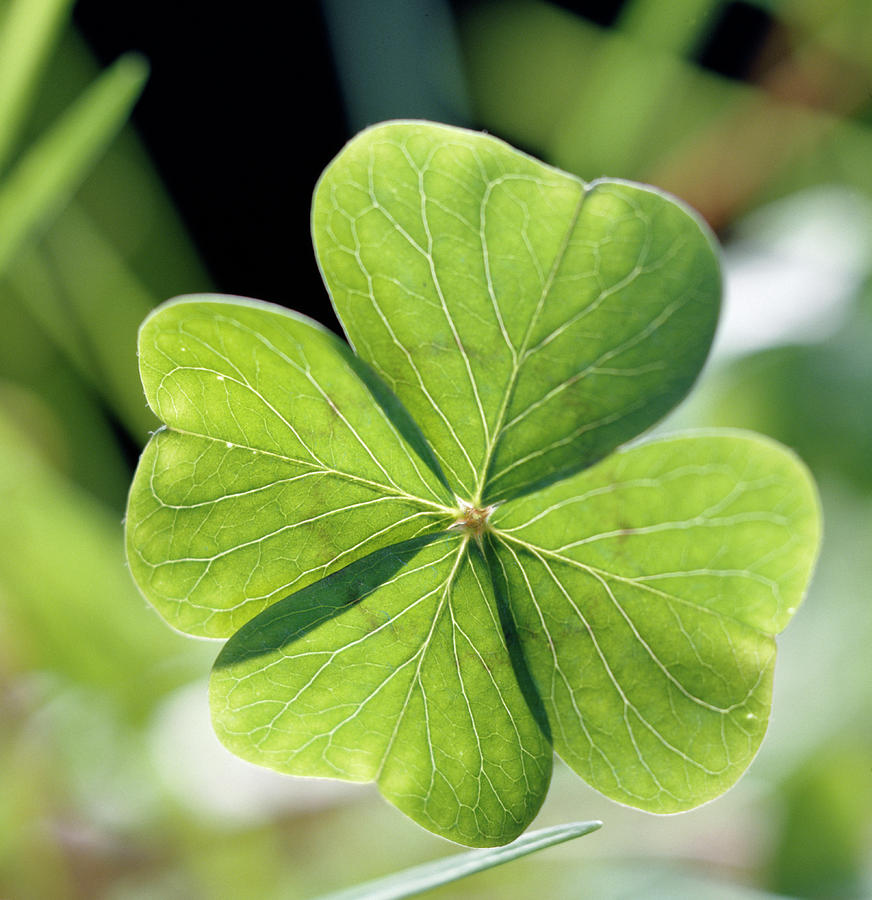This is a detailed, close-up color photo of a unique four-leaf clover, prominently centered in the image. Each leaf, resembling a heart shape, displays a vibrant green color with intricate veins that are white, extending outwards from the star-shaped center where all four leaves meet. The veins have a slightly darker ring or glow around them, highlighting their structure. The background of the photo is blurred, ensuring the four-leaf clover remains the focal point. The entire scene is captured in daylight, emphasizing the natural beauty and distinct features of the clover.